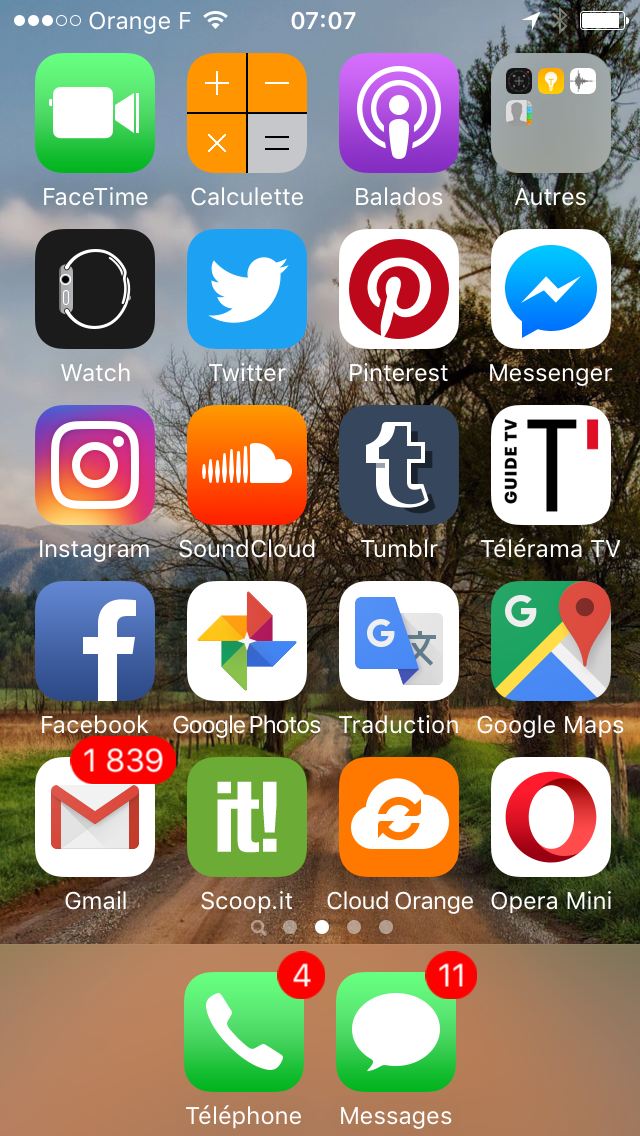Screenshot of an iPhone Home Screen

The screenshot captures the home screen of an iPhone, organized in a 4x5 grid of application icons. At the top left corner, the status bar indicates the carrier "Orange F" with a 70% battery remaining, suggesting it might have been taken in the early evening or later.

The top row of app icons includes:

1. FaceTime
2. Calculator
3. Photos
4. Watch

Continuing down the screen, the subsequent apps appear as follows:

- Twitter
- Pinterest
- Messenger
- Instagram
- SoundCloud
- Tumblr
- Telerama TV
- Facebook
- Google Photos
- Traducción (Translation)
- Google Maps
- Gmail
- Scoop.it
- Cloud Orange
- Opera Mini
- Telephone
- Messages

Notably, the "Telephone" app displays four missed calls, and the "Messages" app indicates 11 unread messages, implying that the iPhone owner is quite active and possibly popular. The wallpaper is understated and provides a neutral backdrop, allowing the colorful app icons to stand out clearly.

Overall, the image showcases a well-organized and functional home screen with a mix of social media, productivity, and utility applications.